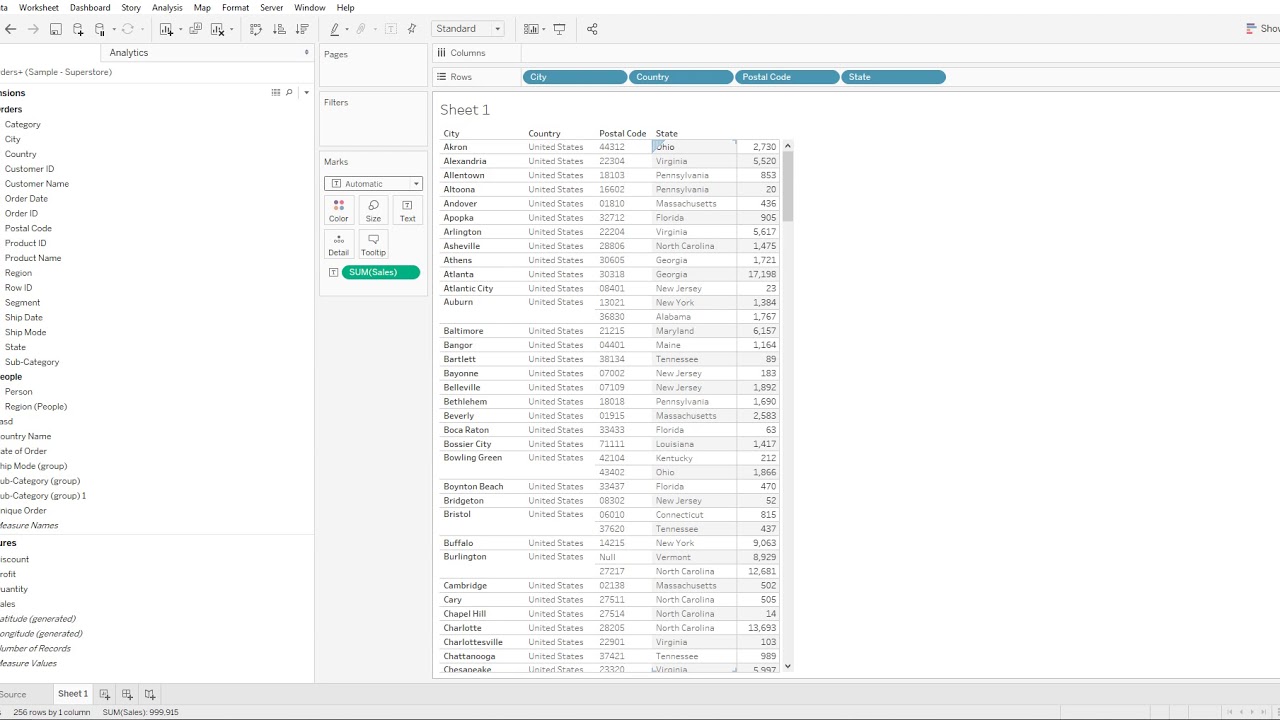The image depicts an application interface, likely a data analytics or visualization tool, with a layout approximately one and a half to two times wider than it is tall. The top section features a horizontal menu bar underlined in white with black text. The menu options include: Worksheet, Dashboard, Story, Analysis, Map, Format, Server, Window, and Help. Below the menu bar, a gray toolbar spans the width of the image, housing navigation buttons such as Back and Forward, followed by numerous icons extending halfway across the screen.

On the left side, a vertical pane with a white background contains a dropdown menu where "Analytics" is selected. Beneath this, there are various selectable metrics, each labeled with succinct terms like Order ID, Product ID, Region, Segment, Ship Data, and more, totaling around 25 items from top to bottom.

Adjacent to this pane, a narrower column provides additional buttons labeled with terms like Pages, Filters, and Marks for further data manipulation and customization.

The main section of the screen, occupying the remaining space, displays a large workspace titled "Sheet 1," which resembles a spreadsheet, likely used for organizing and analyzing data visually akin to an Excel sheet.